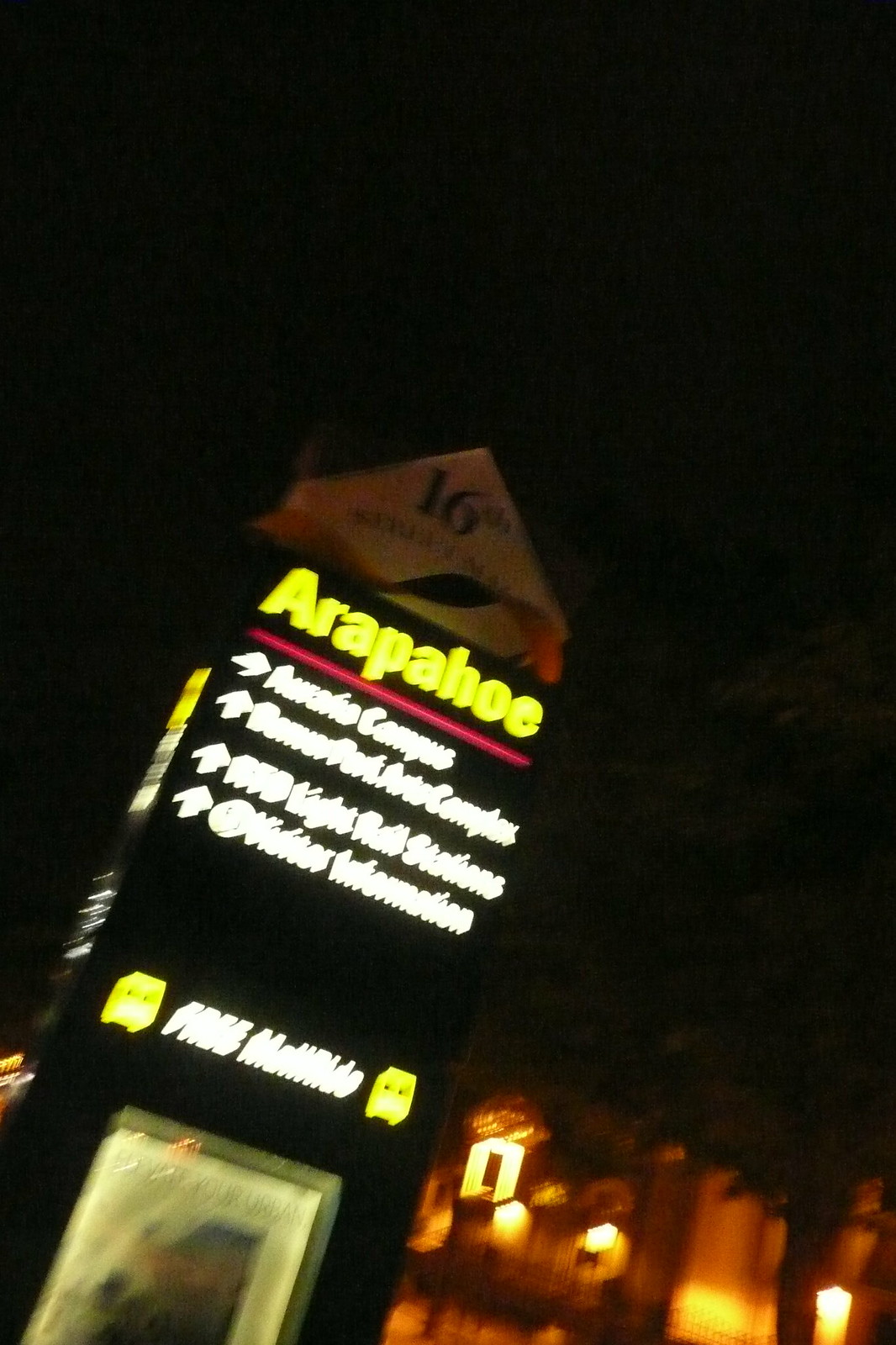Captured at night from inside a car, this image displays a slightly blurry street sign against a backdrop of illuminated trees and a building. The sign prominently features a white triangle at the top, labeled "16th." Below the triangle, the larger text reads "Arapaho," while smaller, less discernible words provide directions to various locations. Clearly visible directional arrows point towards a campus, a light rail station, and a visitor information center. The overall scene hints at a possible light rail station area, with urban elements subtly illuminated in the background despite the blur, creating a night-time urban ambiance.